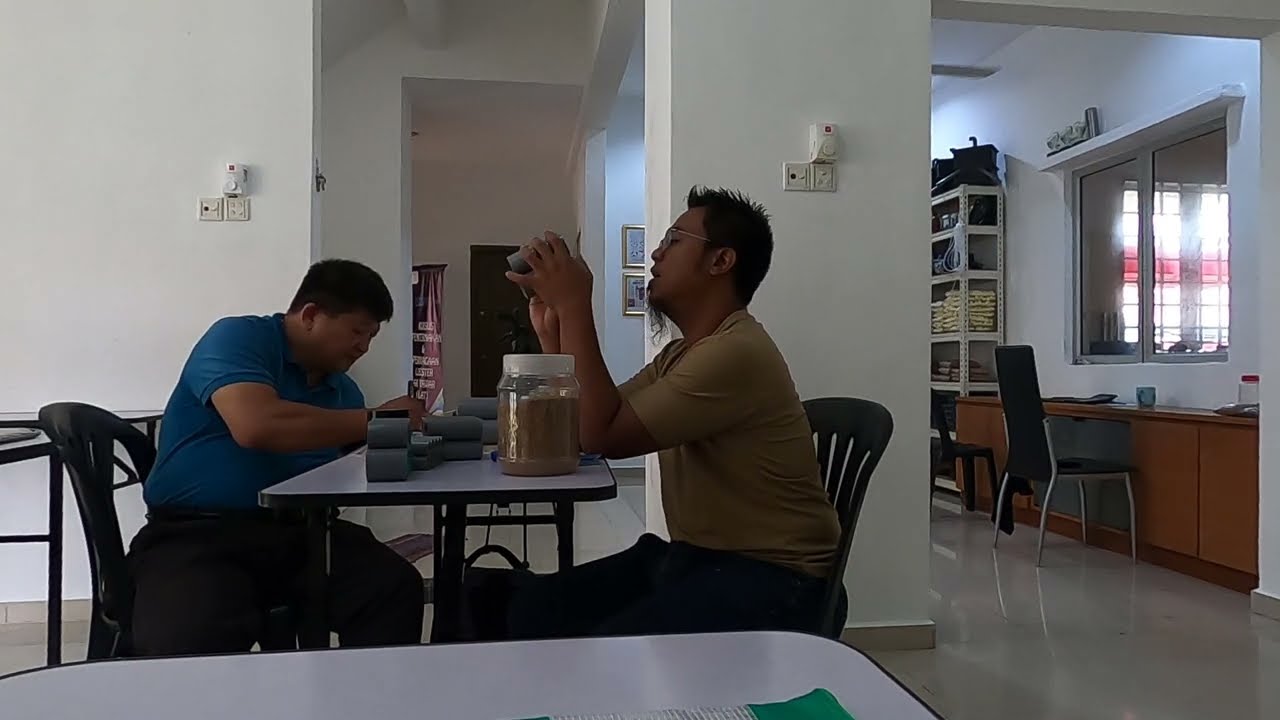The image depicts an indoor office or facility space featuring two men of probable Asian descent seated across from each other at a white table. Both men have dark hair, with the man on the right wearing glasses and a beard, dressed in a beige shirt and black pants, while the man on the left dons a blue shirt and black pants. They are engrossed in a task involving a gray object, though the exact nature of their work is unclear. The table also holds a clear jar containing a brown substance. Both men are seated on black plastic chairs. Surrounding the central table, other unoccupied tables can be seen, suggesting a larger work area. To the right, there is a window and a separate brown desk paired with a black chair. The room is brightly lit, and in the background, a rack displays folded clothing or materials. No other individuals are present in the image, which is rendered in color.